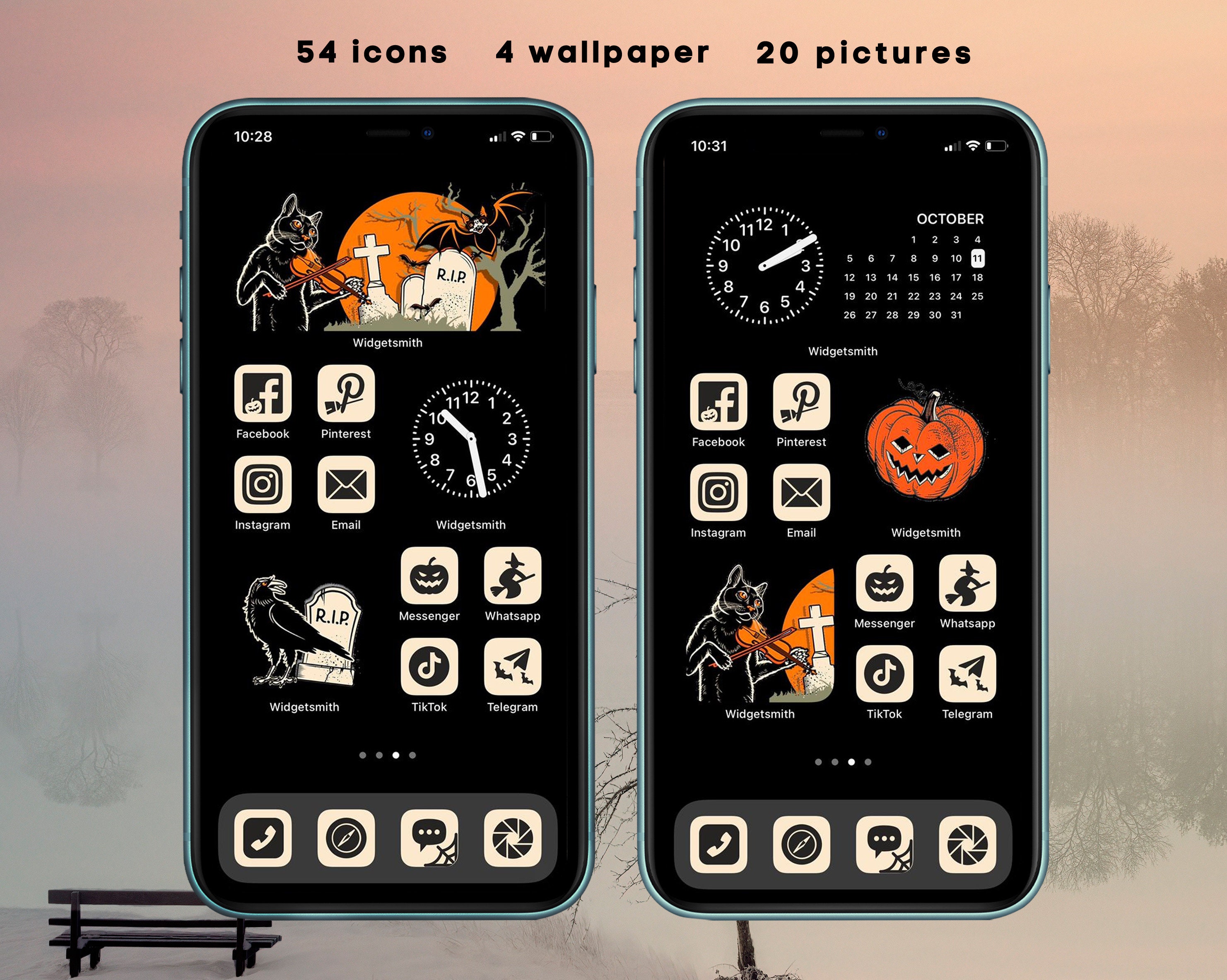This image is a screenshot, likely from an advertisement or website, promoting themed mobile phone wallpapers. It features two smartphones side by side, each displaying different, but similarly styled Halloween-themed backgrounds. The backdrop of the overall image is a pink-toned outdoor scene with a park bench situated in the left corner, under a sky that blends shades of pink, gray, and blue, enhancing the promotional aesthetic.

On the left phone, the background predominantly showcases a spooky graveyard scene under a haunting pumpkin moon. The graveyard imagery includes "Rest in Peace" tombstones, contributing to the eerie Halloween atmosphere. The apps on this phone, such as Facebook and Instagram, are displayed with black and white icons, which resonate with the dark, spooky theme.

The phone on the right mirrors this aesthetic with its own graveyard-themed wallpaper. This background includes a pumpkin moon, a black cat playing a fiddle near a cross-marked grave, and various Halloween-themed elements. The icons on this phone are also black and white, maintaining visual consistency. Notably, the calendar widget at the top of the screen displays the date October 11th, reinforcing the Halloween theme.

The combination of these elements – the pink scenic background, and the detailed, themed wallpapers on the phones – effectively creates a compelling Halloween promotional display.